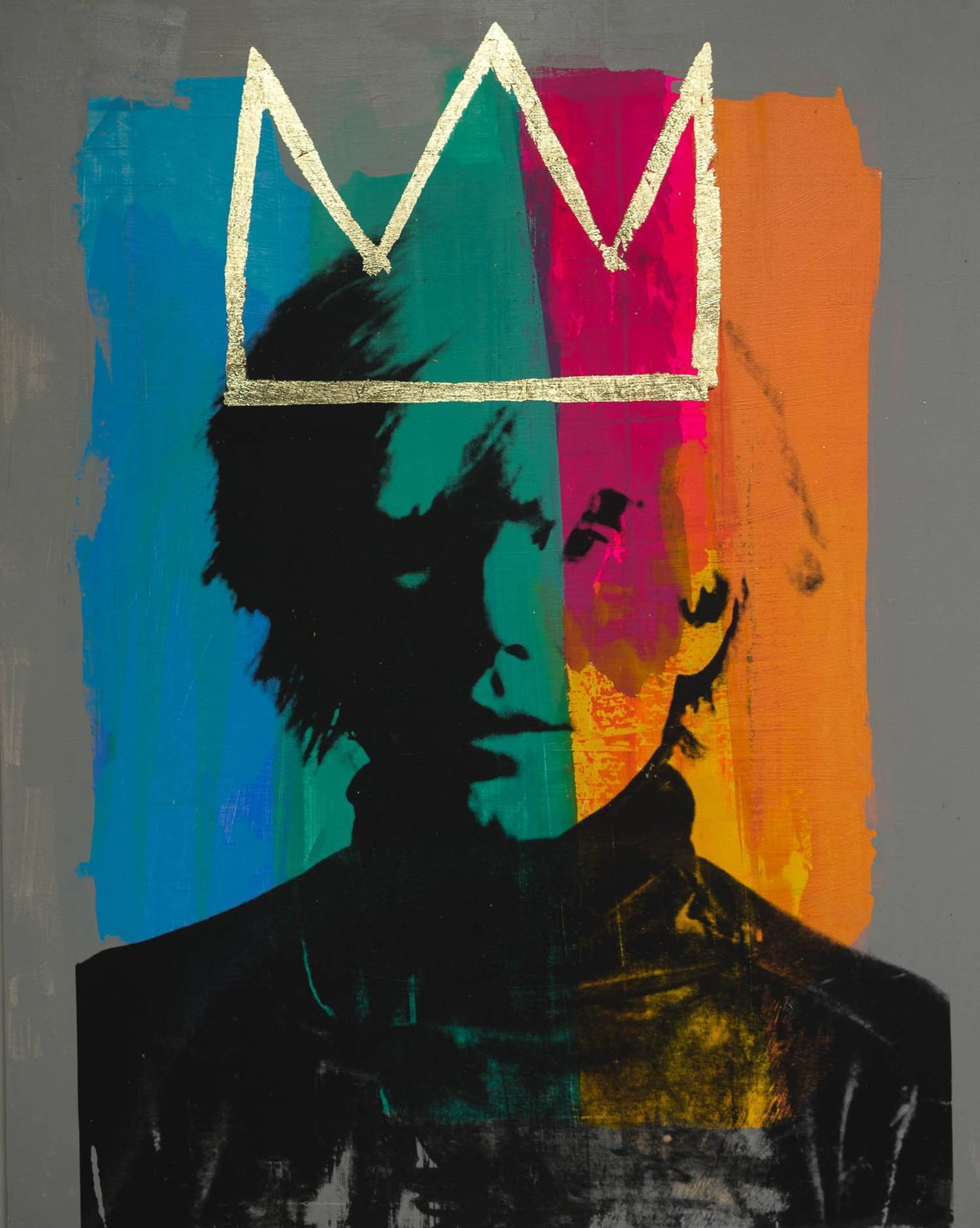The image is a mixed medium painting of the artist Andy Warhol. The background of the painting is predominantly gray, overlaid with four large vertical paint strokes: blue with hints of green to the left, green in the left center, a vibrant pinkish-red transitioning into yellow with spots of orange in the right center, and orange to the far right. Andy Warhol's face is rendered in a stencil style, with the left half of his face painted green, the upper right half pink, and the lower right half yellow. The light areas of his face and hair allow the background paint strokes to show through. Warhol’s black or gray spiky hair stands out, and he appears to be wearing a black turtleneck or suit coat. A simple metallic three-pointed crown, seemingly drawn with a paint marker, adorns his head, further emphasizing his iconic status.